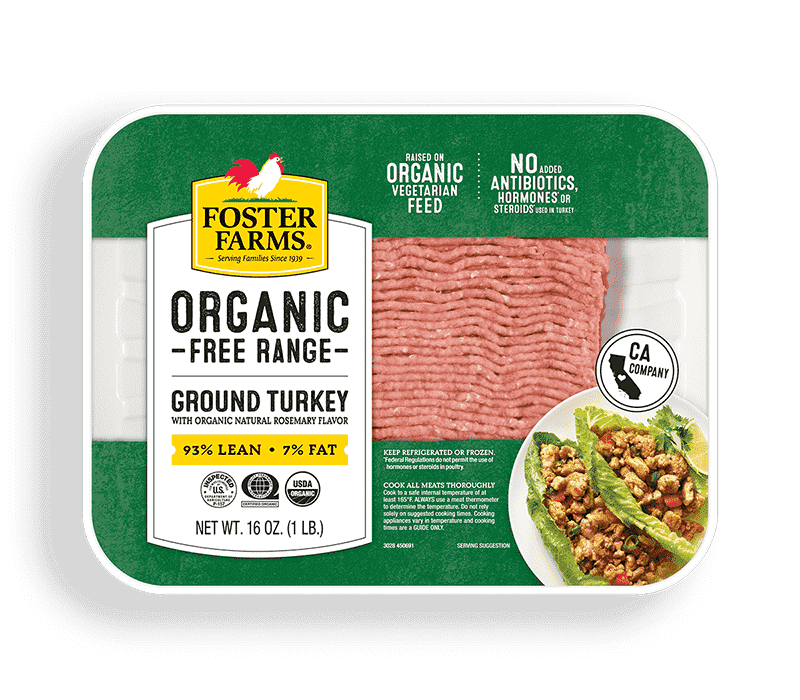The image displays a top view of a package of organic free-range ground turkey, likely packaged in a white styrofoam or plastic base covered by a labeled, clear plastic wrap. The package features green borders at the top and bottom, with white text on the top border stating "raised on organic vegetarian feed, no added antibiotics, hormones, or steroids used in turkey." The bottom green band includes storage and cooking instructions. On the right side of the package, there is a white circle with black letters reading "CA Company," accompanied by a black outline of California with a white heart in the center. Just below, there is an image showing a serving suggestion of ground turkey wrapped in large lettuce leaves with minced vegetables. To the left, on a yellow background, the brand name "Foster Farms" is prominently displayed with the tagline "Serving families since 1939," along with an emblem of a white rooster with a red comb and wattle. Below this, on a white background, the product details read "Organic Free-Range Ground Turkey with Organic Natural Rosemary Flavor, 93% Lean, 7% Fat," with the net weight noted as "16 ounces (1 pound)."